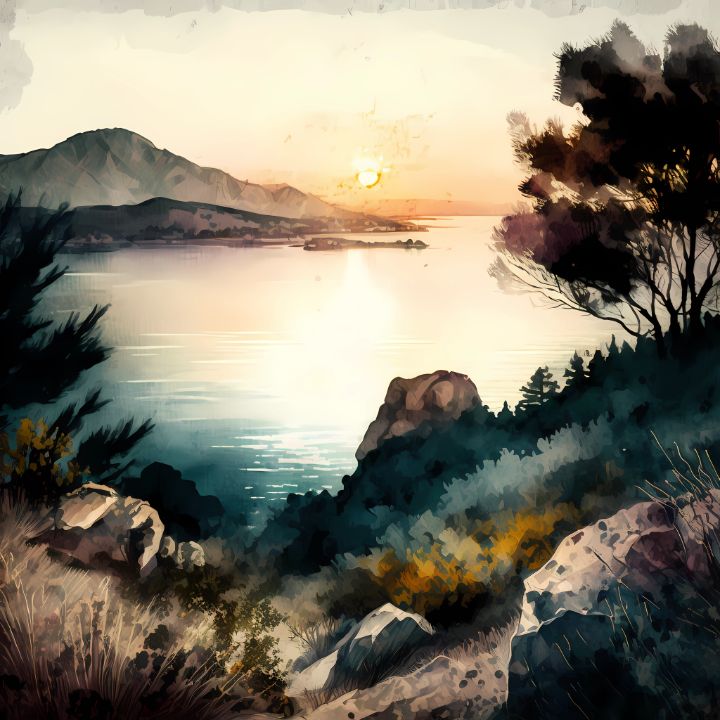The image is a detailed watercolor painting, possibly with hints of digital enhancement, depicting a serene lakeside scene during a sunset. In the foreground, there are sizable gray rocks and lush green foliage, including a mixture of bushes and trees. The trees vary in shape, with some having bushy, round tops and others appearing more like silhouettes with long leaves. The foreground vegetation also includes patches of brownish and bluish grass, and clusters of yellow flowers.

The calm lake, reflecting the setting sun, stretches across the middle of the scene, forming almost a V-shape that guides the eye towards the background. Here, the water's surface captures hues of pink, orange, and green, enriched by the warm, dim light of the sunset. The sun itself is a small, brilliant spot of white-yellow near the horizon, casting a soft glow across the scene.

On the opposite shore, the landscape rises into hilly elevations that transition from green closer to the lake to grayish as they ascend into a mountain range. The mountains, painted in shades of gray and white, appear somewhat abstract and merge gently with the skyline. The sky is a gradient transitioning from a soft white at the top to shades of pink, orange, and yellow nearer the horizon, complemented by a few clouds lingering on the left side.

Overall, the image employs a palette of dark and muted tones—grays, blues, purples, and browns—counterbalanced by the vivid colors of the sunset and the occasional spots of yellow and pink in the vegetation. The composition evokes a peaceful and contemplative atmosphere, rich in natural beauty and subtle detail.